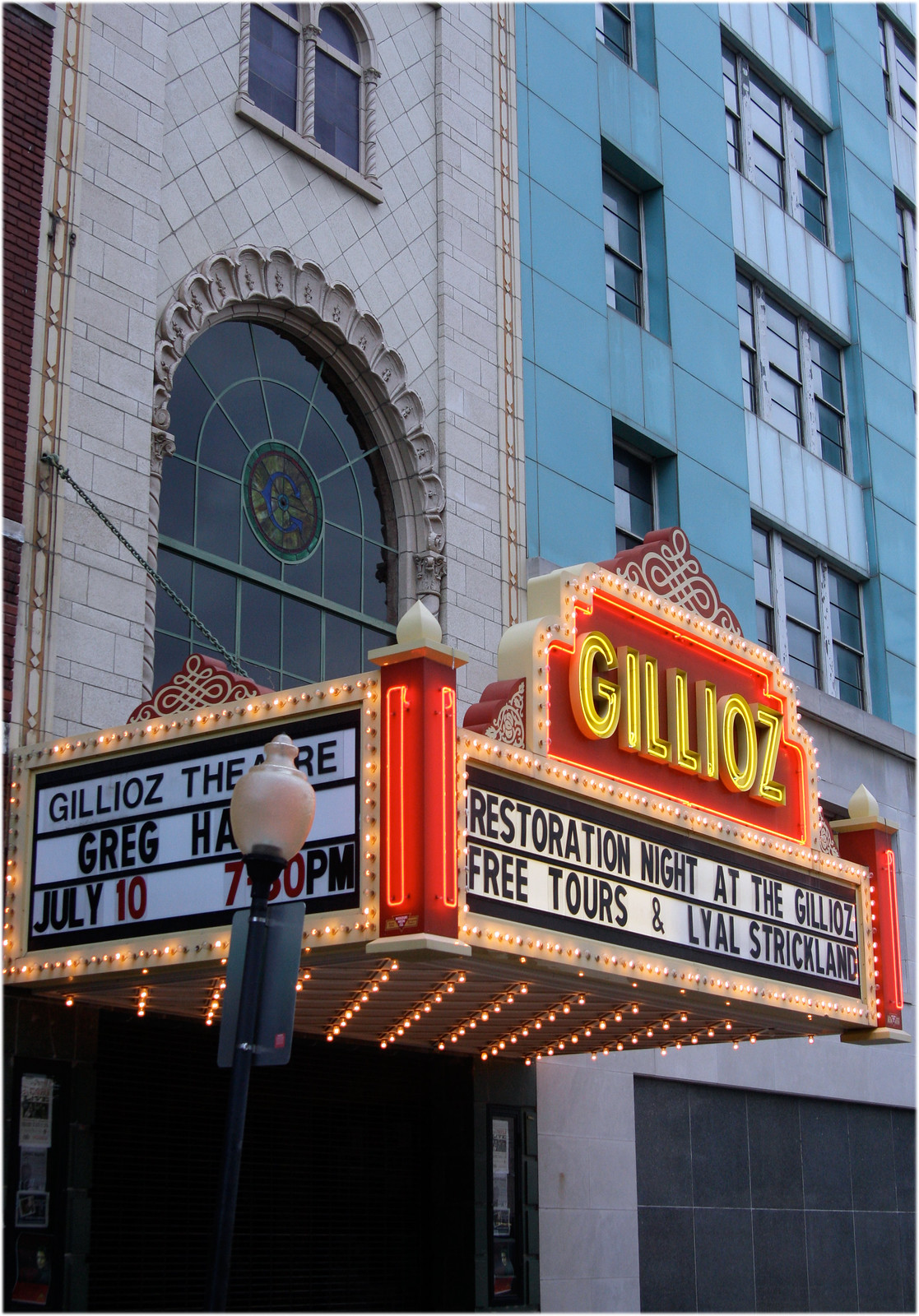This color photograph captures the vibrant and ornate marquee of the historic Gillioz Theater. The tan stone building with an adjoining blue building featuring large rectangular windows evokes the architectural charm of cities like New York or Chicago. The marquee, illuminated with bright lights, showcases a red background with neon yellow lettering that spells out "GILLIOZ." The white marquee below, adorned with black capitalized text, announces "Restoration Night at the Gillioz," offering "Free Tours" and a performance by "Lyle Strickland." A partial street lamp obscures part of the sign, revealing "Greg H.A." along with the details, "July 10th," and "7:30 PM." The entrance, glowing warmly, resembles that of a classic theater or movie house, adding to the photograph's nostalgic feel.